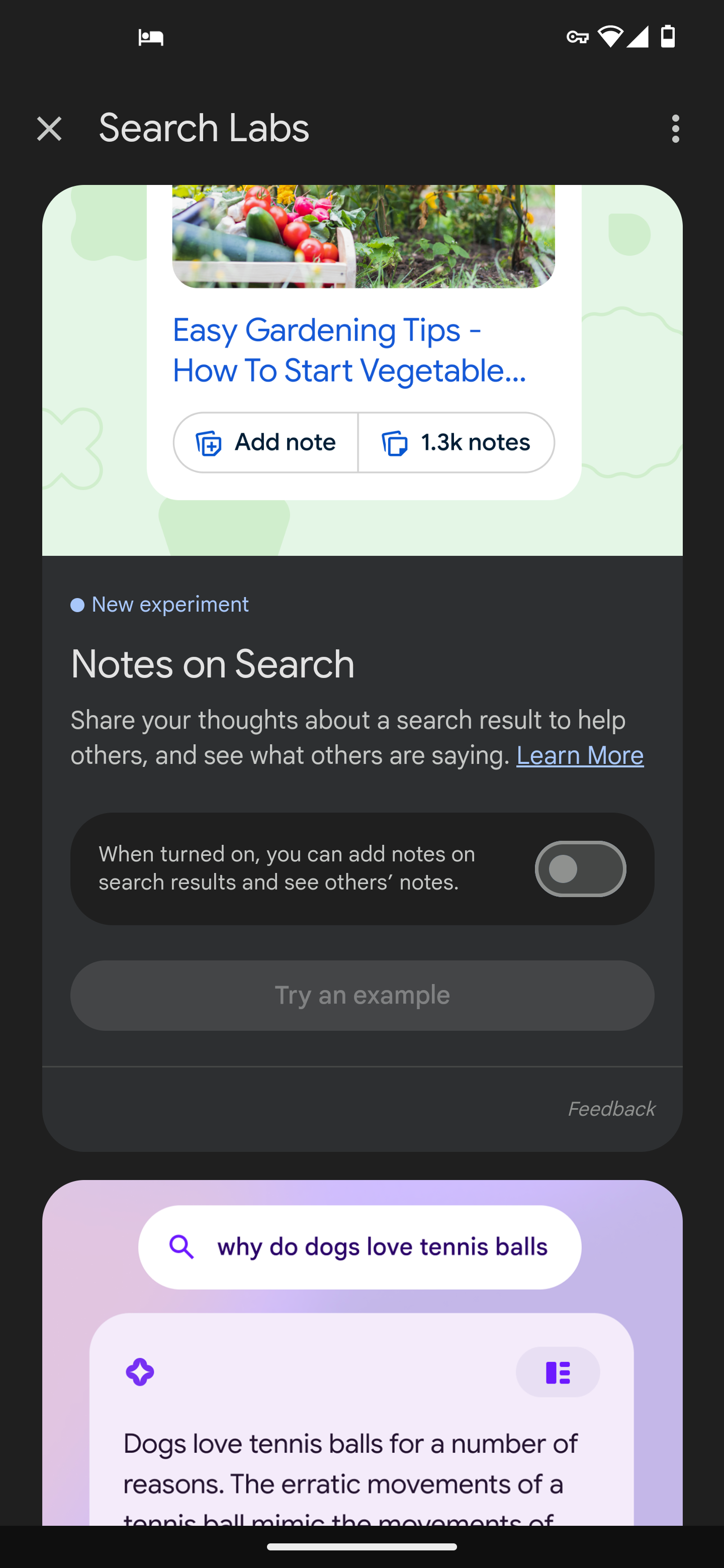This screenshot, captured from a phone set in dark mode, showcases a search result page with various elements visible. The battery icon at the top right indicates it's nearly half charged, while full service strength and Wi-Fi connectivity are also observed. Along the top row of text, "Search Labs" is displayed next to an 'X' button to close, and on the far right, a three-dot drop-down menu.

The primary image within the screenshot is partially visible but appears to show vegetables in a container with leafy plants in the background, hinting at a gardening theme. The headline adjacent to the image reads, "Easy Gardening Tips: How to Start Vegetables." There is also an option to "add a note," and it is noted that 1.3K notes have already been added.

Beneath this, a section titled "New Experiment Notes on Search" explains the feature: "Share your thoughts about a search result to help others and see what others are saying. Learn more. When turned on, you can add notes to search results and see others' notes. Try an example." The example given hints at a popular search query, "Why do dogs love tennis balls?" However, the text cuts off after beginning to explain with, "Dogs love tennis balls for a number of reasons. The erratic movement of a tennis ball mimic the movements of..."

Overall, the screenshot provides a glimpse into search innovations and user interactions, emphasizing the integration of community feedback through comment-like notes.